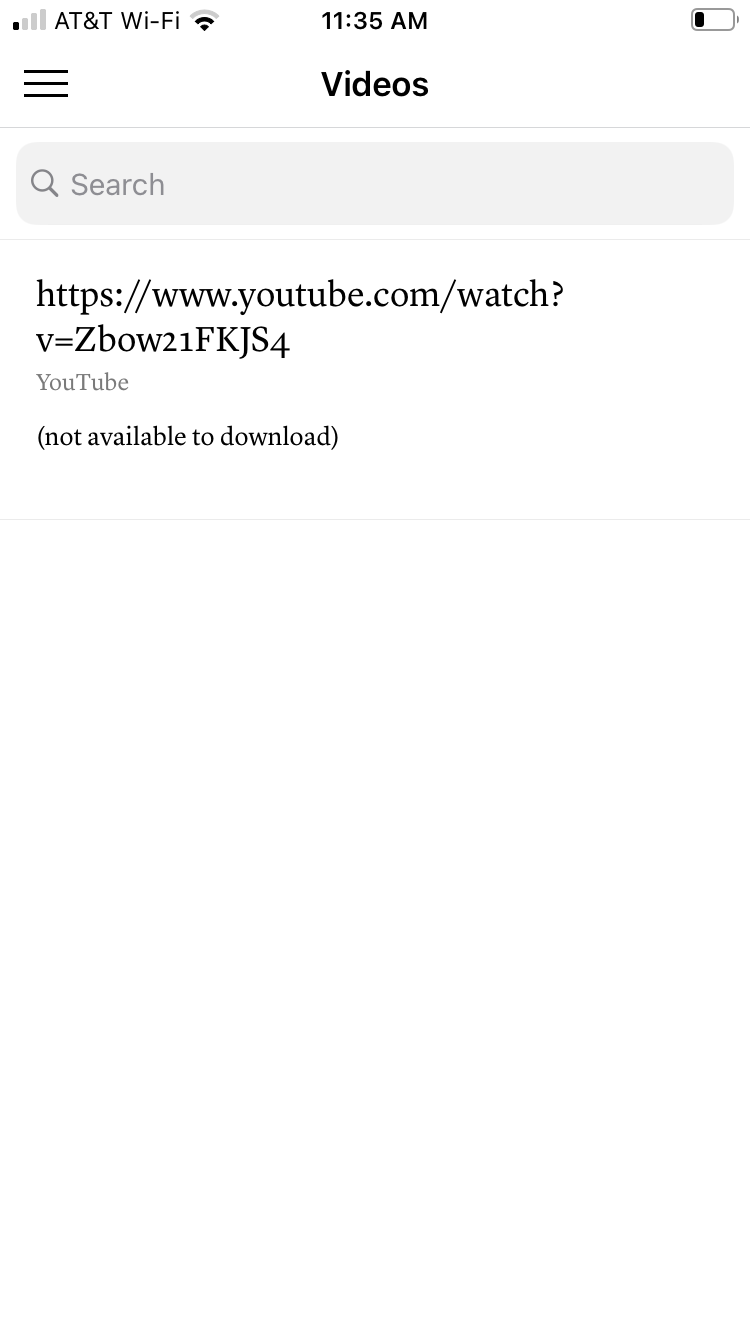The image displays a multitude of interface elements, predominantly presented in shades of gray. On the top left-hand side, there are four vertical bars of varying height, starting with the shortest dark gray bar and progressively taller lighter gray bars. To the right of these bars, the text "AT&T" and "Wi-Fi" are visible alongside the Wi-Fi signal icon. Centrally aligned at the top, the current time is displayed as "11:35 AM". Adjacent to this, a battery icon is shown containing a small gray rectangle inside, indicating the remaining charge.

Beneath the initial setup on the left-hand side, there are three horizontal bars stacked vertically. In the middle of the image, the word "Videos" is prominent, followed by a thin gray line underneath it. Continuing downward, there is a gray rectangle featuring a magnifying glass icon and the word "Search".

The next segment includes a URL starting with "https://www.youtube.com/watch?", followed by a unique identifier: "B=Zbow21fkjS4". Below this, the word "YouTube" appears, with a note in parentheses stating "(not available to download)". A light gray line separates this section from a vast area of blank white space beneath it. This comprehensive description encompasses all elements visible in the image.